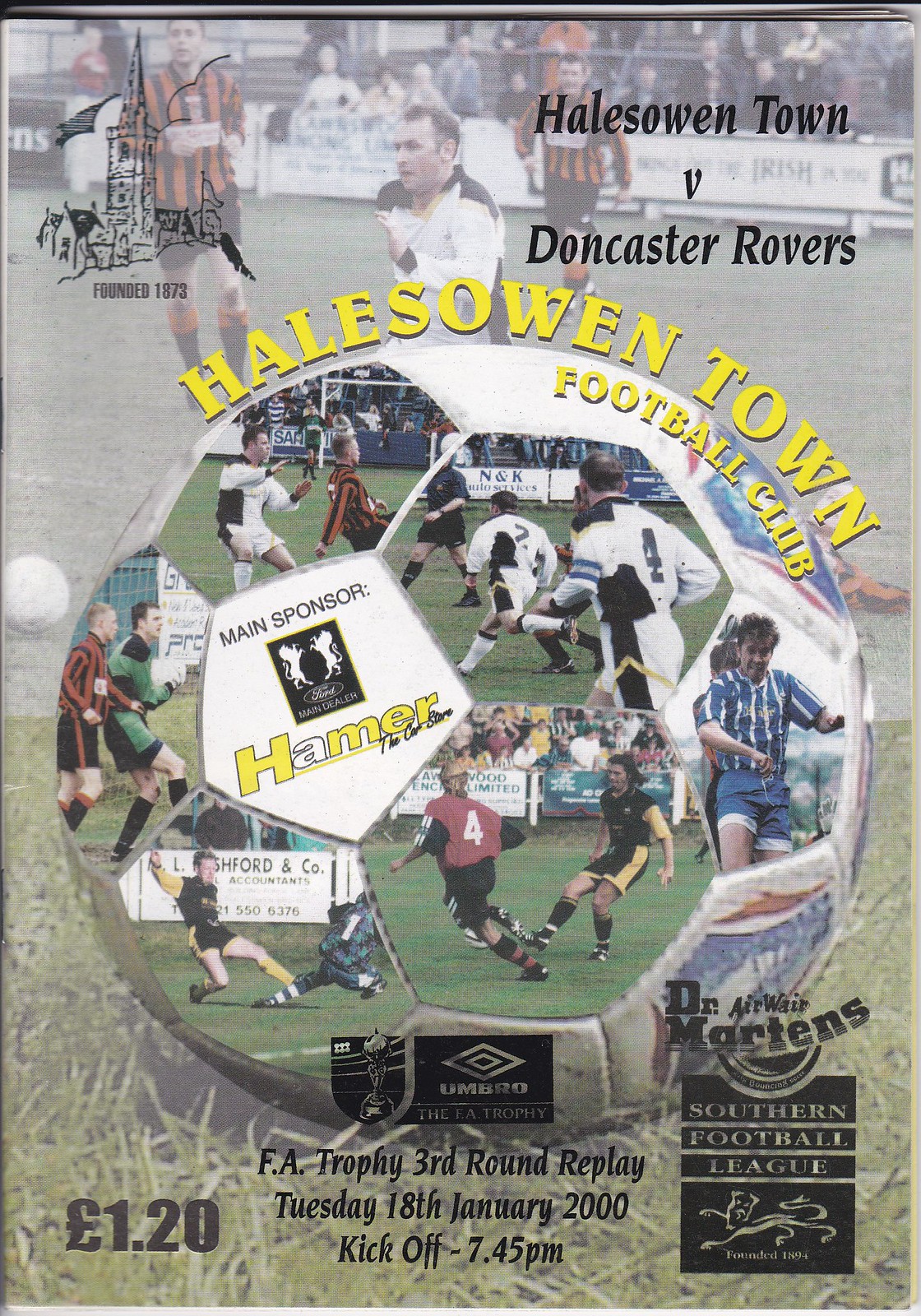In this vertically long, heavily modified photograph, a central soccer ball rests on a grassy field surface, occupying the lower portion of the image. The soccer ball is unique, as each of its hexagonal tiles contains separate images of soccer matches. The grassy field surface transitions halfway up the image to a lighter gray background displaying a dynamic scene of soccer players in action. Surrounding the soccer ball is an amalgamation of text and additional imagery. 

At the top right, black text announces a match between "Hailstown versus Doncaster Rovers," while to the left, an illustration of a castle is accompanied by the founding year "1873." Encircling the ball, the words "Hailstown Football Club" appear in bold yellow text. The standout hexagonal tile on the soccer ball displays the main sponsor information: "Ford, Hammer, the card store." Below the ball, additional text provides event details: "Umbro to FA Trophy, FA Trophy third round replay, Tuesday, 18 January 2000, kickoff 7:45 PM." The bottom left corner indicates the original price, "£1.20," and the bottom right corner features branding for "Dr. Marten's Airwear, Southern Football League." The image masterfully combines visual elements of a soccer game with promotional and event-specific information, creating an intricate and engaging composite.